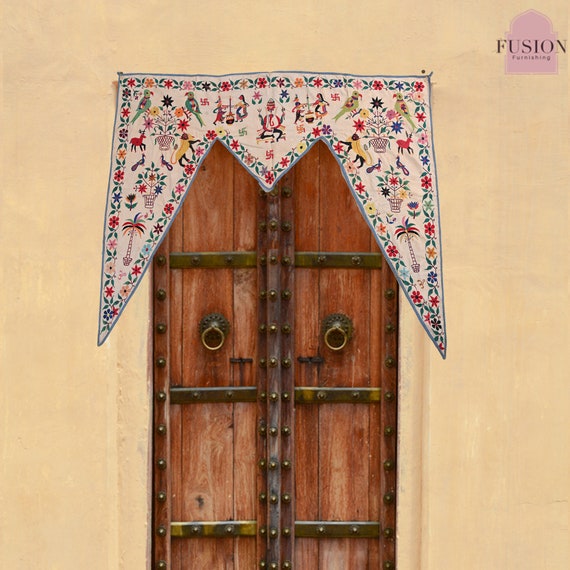The image depicts a wooden double door set within a pale yellow, possibly tan wall that might be concrete or dried mud. Each door features black metal handles and brass knockers adorned with circular designs. The framework of the doors includes brass metal with rivets, adding a decorative element above and below the door knockers. A prominent embroidered or quilted curtain, patterned with animals and flowers and bordered with floral designs, drapes over the doors. The curtain has a gray outline and hangs in an M shape, with elongated triangular tips on the sides and a shorter triangular tip in the center. In the upper right corner, there is a business logo resembling a badge with a Middle Eastern dome shape at the top. The logo reads "FUSION FURNISHING" in all caps, with a pink background behind the lettering.